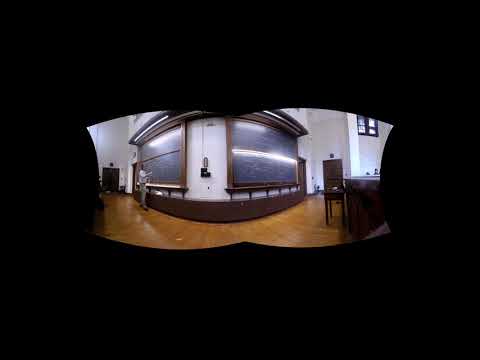A black border frames the image, focusing on a brightly lit rectangular area at the center, depicting a classroom or lecture theater. The scene features two large blackboards with noticeable wooden trim along their edges. White chalk marks are visible on both boards. The wall curves into a semicircle or arch and is primarily white, with a wooden panel running horizontally along the bottom. 

On the left side of the image, a man in beige pants and a white shirt stands near one of the blackboards, appearing to write or work on it. The floor is a light hardwood color, adding warmth to the scene. In the background, we can see multiple doors – two on each side of the room. A wooden strip runs beneath the boards, and to the left, a long table with a small shelf is visible. The ceiling is also white, complementing the walls. The bottom part of the image reveals a bit of seating area, possibly the first row of student seats, suggesting an educational setting.